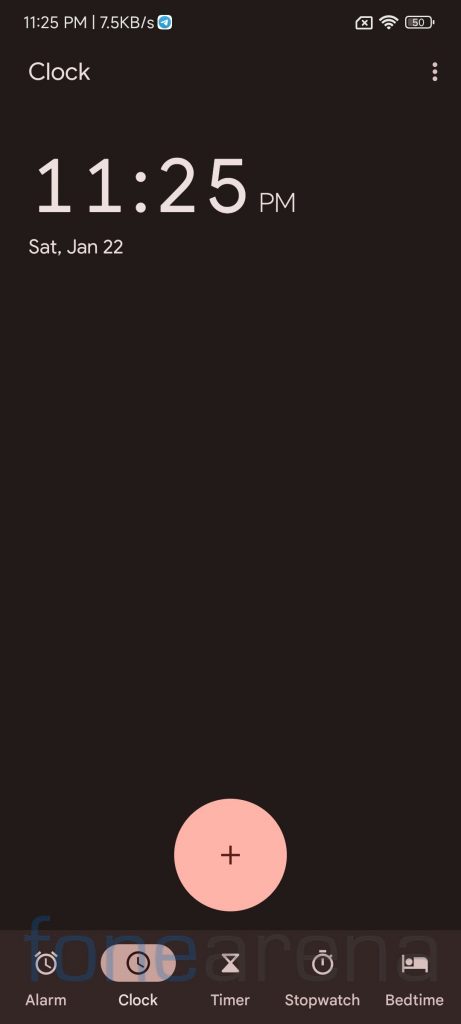The image is a screenshot from a cell phone with a completely black background. At the top, in white text, it displays the time "11:25 p.m." Below the time is a horizontal line, followed by the data transfer rate "7.5 KB/s". Additionally, there is a small white square with soft, rounded edges. Within the square, there's a blue circle featuring an icon resembling a paper airplane, pointing between the 1 and 2 o'clock positions, symbolizing a sent message.

To the right of the blue circle icon, there is a series of small icons: a SIM card icon with an 'X' inside (indicating no SIM card or no network), a Wi-Fi signal icon, and a battery icon displaying "50", indicating 50% battery life.

On the top left side of the screen, the word "Clock" is written in thin, white capital letters. On the top right side, there are three vertical dots, typically representing a menu or settings option. The time "11:25 p.m." is prominently displayed again in larger white text, with "SAT Jan 22" underneath it, denoting Saturday, January 22nd.

At the bottom center of the screen, there's a light pink circle featuring a small plus sign inside it, likely a button to add something. Along the bottom edge of the screen are five icons: an alarm clock, a standard clock, a timer, a stopwatch, and a bedtime icon, indicating different clock-related functions available on the device.